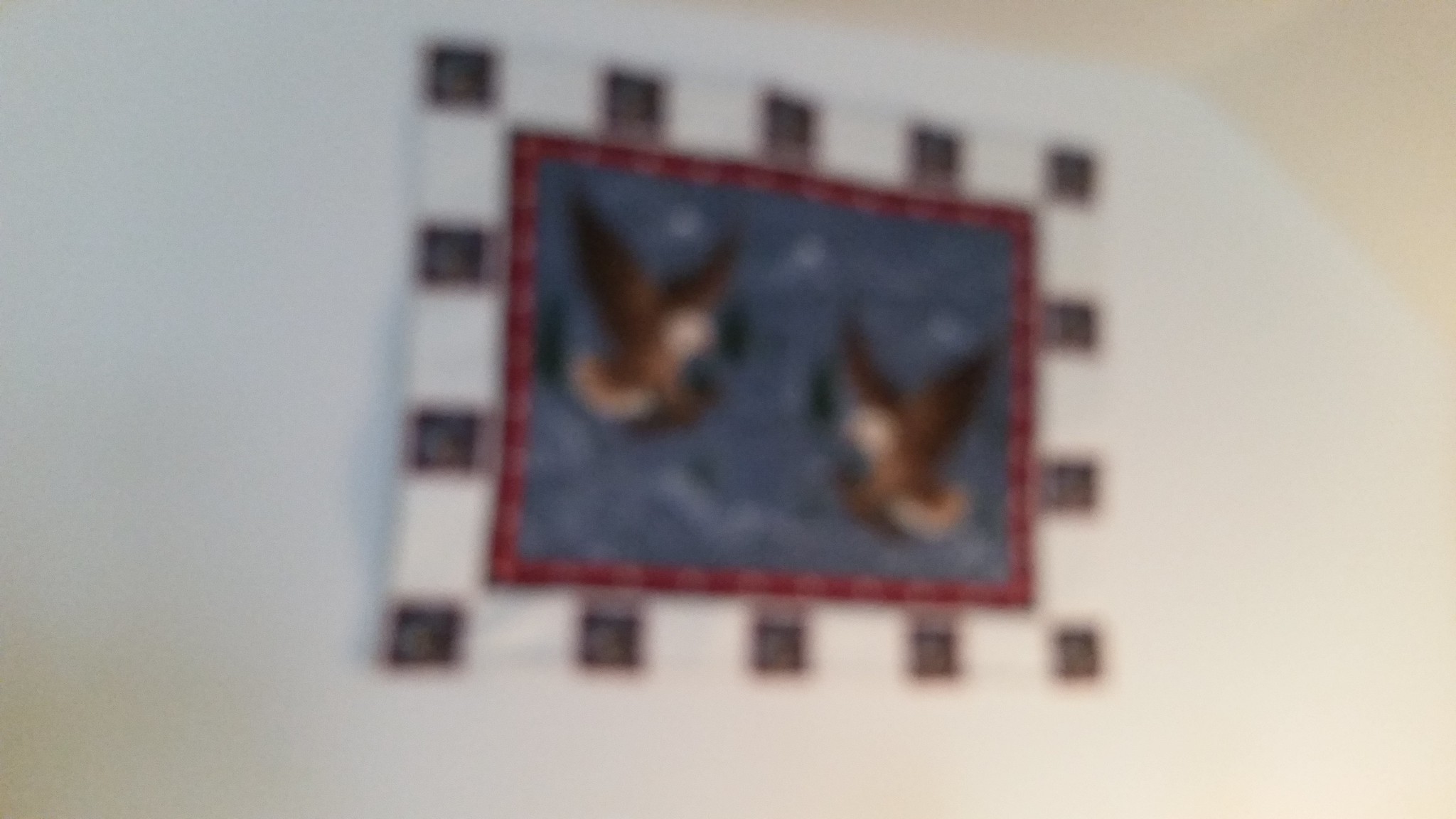This is a very blurry photograph of a piece of artwork hanging on a wall. The artwork has a distinctive border pattern: a white frame adorned with black squares, including a set of squares in each corner, three squares at the top and bottom, and two squares on each side. Inside this border is a reddish-purple or burgundy section. The central image features a blue background with some white dots scattered throughout. Depicted within this blue area are two bald eagles facing each other. One eagle is positioned near the top right, with its wings raised upward, while the other is at the bottom left, also with its wings up and its head facing downward. The wall behind the artwork appears white, though the upper left corner shows a light cream color. Due to the image's blurriness, the details of the eagles and overall artwork are heavily obscured.